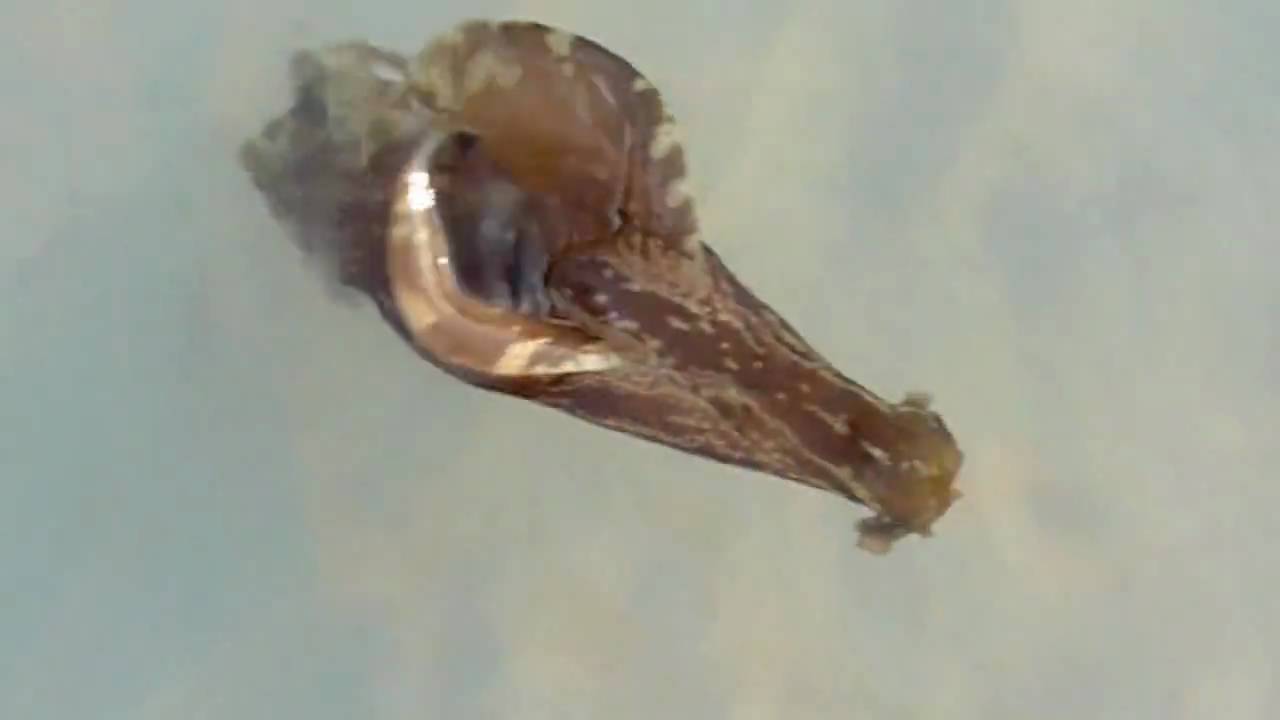This image appears to be an out-of-focus, close-up shot of an unidentified object. The background is a blend of different shades of white and blue, resembling a cloudy sky but somewhat murky and blurred. At the center of the picture, there's an ambiguous shape that some describe akin to a seahorse head or maybe a snail or shell. The object is predominantly brownish with pinkish hues, white stripes, and scattered white dots. The top part of the object displays shades of gray, and the structure's overall form appears to be oval with a long, pointed front reminiscent of a seahorse's head. There is an element of shininess to it, adding to the unclear nature of what exactly it might be. The photograph itself looks old and worn out, contributing to its faded and unappealing appearance.